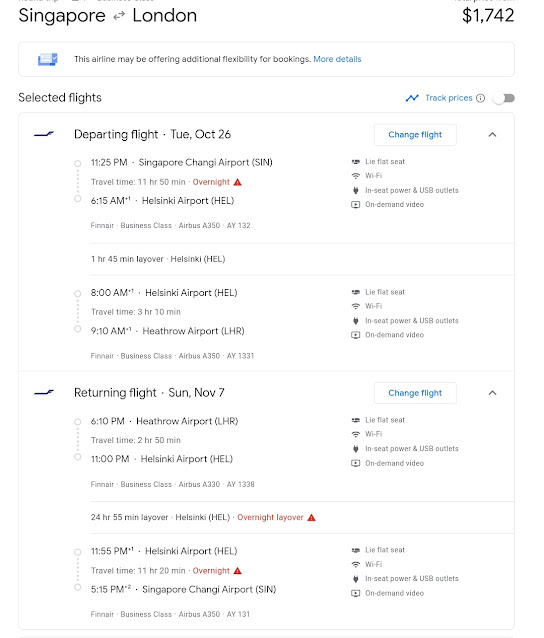This image is a portrait-oriented snapshot featuring detailed flight information for a round trip between Singapore and London. The background is predominantly white with thin grey lines highlighting different text boxes, though no defined border frames the entire image.

In the top left corner, the destinations "Singapore" and "London" are displayed, connected by arrows indicating the round trip nature of the journey. To the right of these destinations, the total fare of $1,742 is prominently shown. 

Directly below, amid some white space, there's a long rectangular, landscape-oriented text bubble outlined in thin grey with rounded edges. This bubble informs viewers that the airline might offer additional flexibility for booking, accompanied by a blue "more details" link.

Further down, the section labeled "selected flights" provides a detailed itinerary. Beside it is a blue link entitled "track prices," all enclosed in a portrait-oriented box with a thin grey border.

At the top of this itinerary box, an icon indicates the departing flight on Tuesday, October 26th. The route from Singapore Airport to Helsinki Airport is detailed, featuring a 1 hour and 45-minute layover in Helsinki before proceeding from 9 AM to 8 AM onward to Heathrow Airport.

For the returning flight, scheduled on Sunday, November 7th at 6:10 PM, the itinerary shows the journey from Heathrow Airport back to Helsinki Airport, followed by an extended layover of 24 hours and 55 minutes, noted as an "overnight layover."